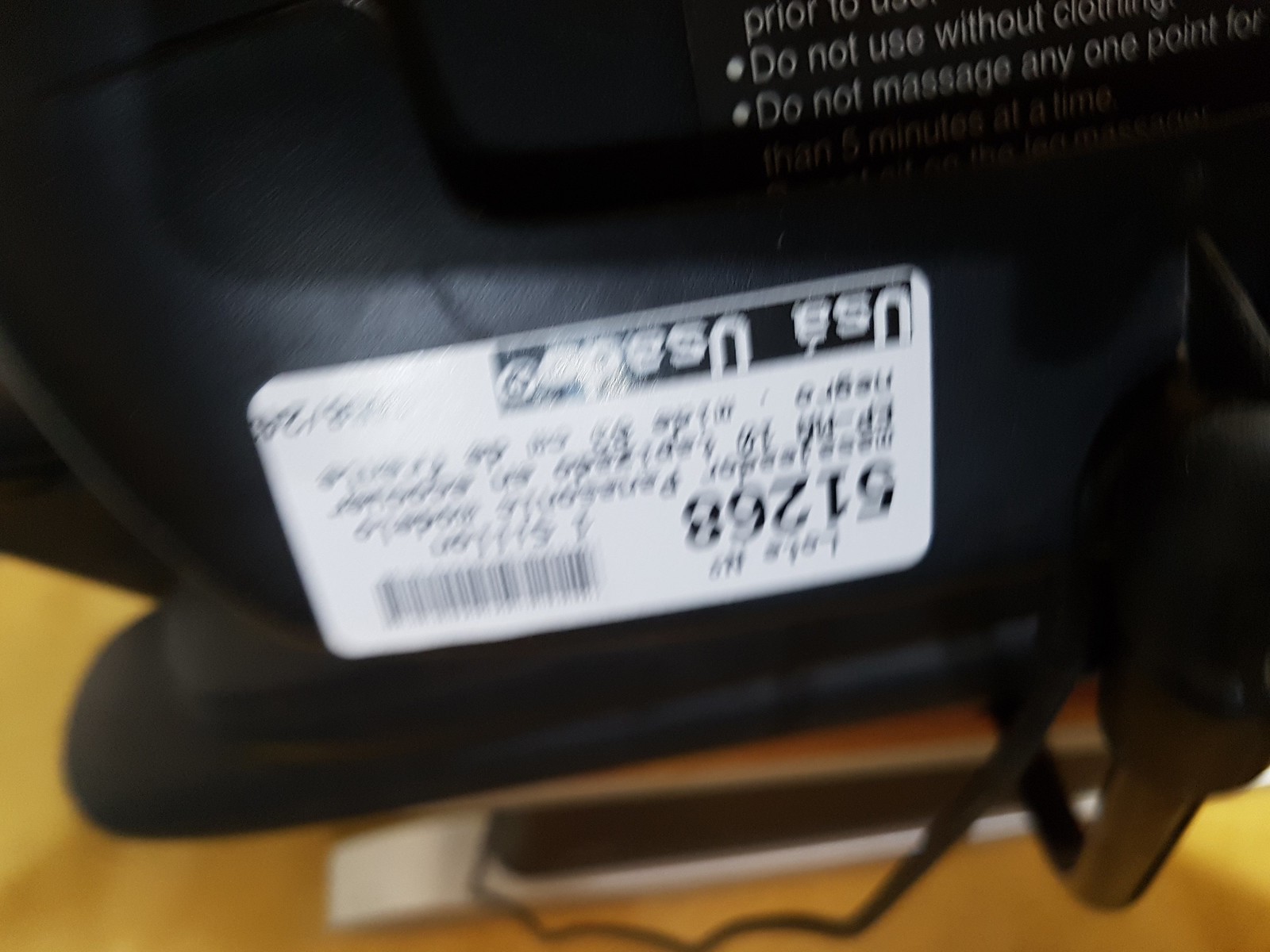In this photo, the bottom half features a yellow background, while the main focal point is a black electronic device, likely a part of a larger object, possibly a power supply or component with a cord running from it. The device displays a prominent, upside-down white label that includes a barcode, the number "51268," and the word "USA." The printing on the label is otherwise too blurry to fully decipher. Additionally, some readable safety instructions printed on the black device itself state "Do not use without clothing" and "Do not massage any one point for more than five minutes at a time." The photo captures only about a fourth of the black device, making it challenging to identify conclusively.